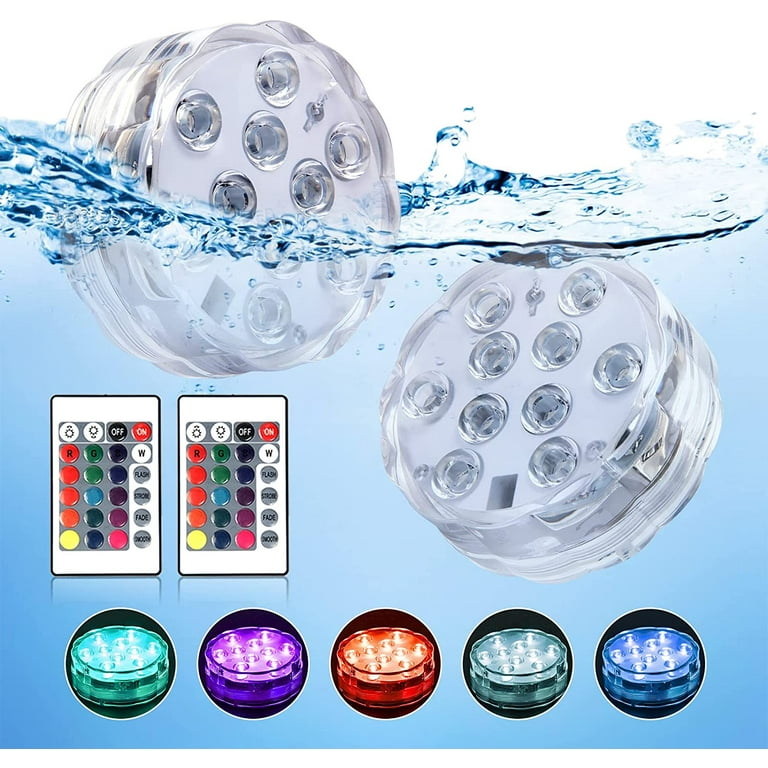This advertisement showcases two cylindrical, clear LED lights that are demonstrated to be water-resistant or waterproof by being partially submerged in water—the left cylinder is half submerged while the right cylinder is fully submerged. Each cylinder has a round face adorned with 10 small LED circles arranged in an X pattern, along with one circle at each side of the round face. At the bottom of the image, there's a display of five different lighting colors emitted by the LED lights: teal (leftmost), purple, red (center), dark teal, and blue (rightmost). 

To the left of the image, a remote control is depicted, featuring a variety of colored buttons. The top left section of the remote houses brightness adjustment buttons (up and down). On the right, it includes a black off button and a red on button, as well as buttons labeled W, flash, fade, and others for various light effects. The image suggests that the set includes two LED lights and two remote controls, each capable of changing the light colors.